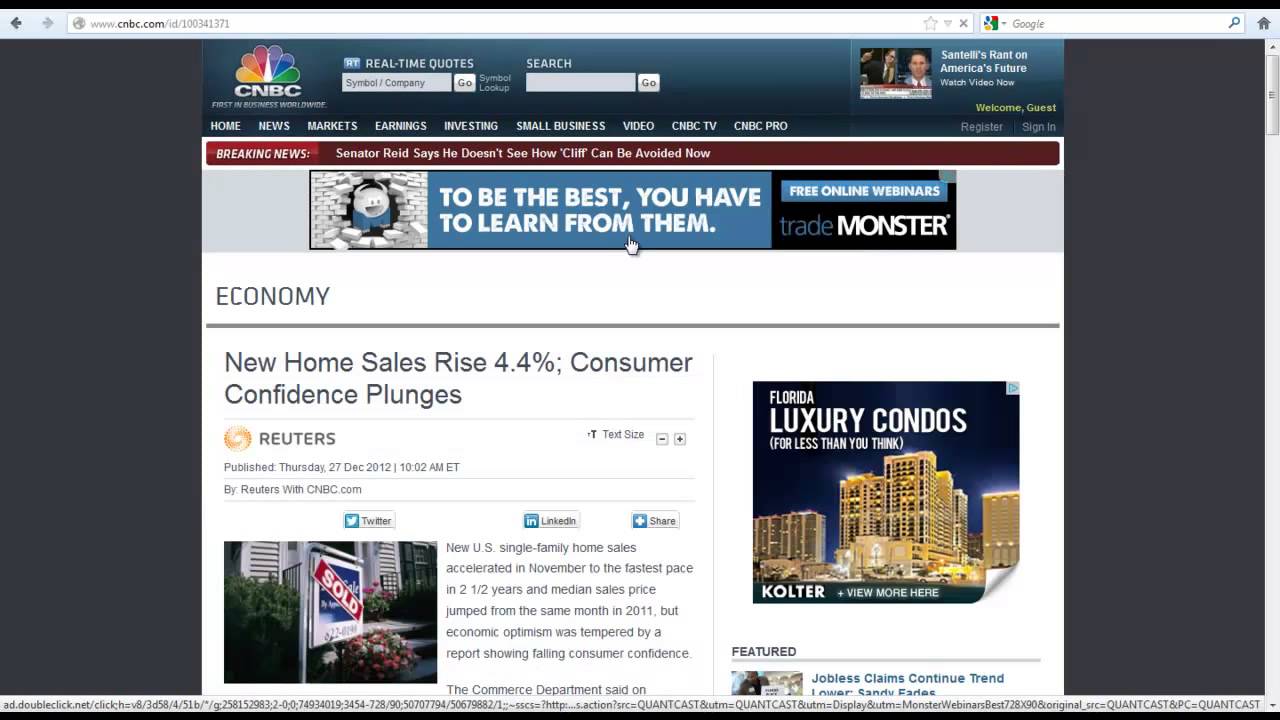The image features a detailed snapshot of the CNBC website displayed on a computer screen. The top of the page prominently showcases the iconic NBC peacock logo above the acronym "CNBC" in bold white letters. The URL bar reads "www.cnbc.com/day/200341372," while adjacent features include a Google search field on the right and a home icon at the far right.

Below the logo, various buttons display real-time financial quotes, where users can enter a company name or symbol in a blank search bar and click "Go." To the right is a headline titled "Santel's Rant on America's Future" with an option to watch the video.

The website's main navigation bar includes links to sections such as Home, News, Markets, Earnings, Investing, Small Business, Video, CNBC TV, and CNBC Pro. On the right side of this bar, buttons for "Register" and "Sign In" are available, with a yellow "Welcome Guest" message above them.

The central content area leads with a "Breaking News" alert, announcing "Senator Reid says he doesn't see how CLIF can be avoided now." Below, a banner ad from Trade Monster promotes free online webinars with the slogan "To be the best, you have to learn from them."

In the Economy section, marked with a solid line, a headline reads "New Home Sales Rise 4.4%; Consumer Confidence Plunges," attributed to Reuters. The detailed breakdown reports that U.S. single-family home sales surged in November to their fastest pace in two and a half years, with median sales prices significantly higher compared to the same month in 2011. However, this optimism is dampened by a decrease in consumer confidence, a piece beginning with "The Commerce Department said on." The report is timestamped Thursday, 27 December 2012, at 10:02 a.m. Eastern Time, and authored by Reuters in collaboration with CNBC.com.

Adjacent to the main article, a right-side advertisement for luxury condos in Florida, marketed as more affordable than anticipated, features a view of tall apartment-style buildings with the brand "KOLTER" and an invitation to "View More."

Further to the right, a featured article headline reads "Jobless Claims Continue Trend Lower," providing easy access to additional related content.